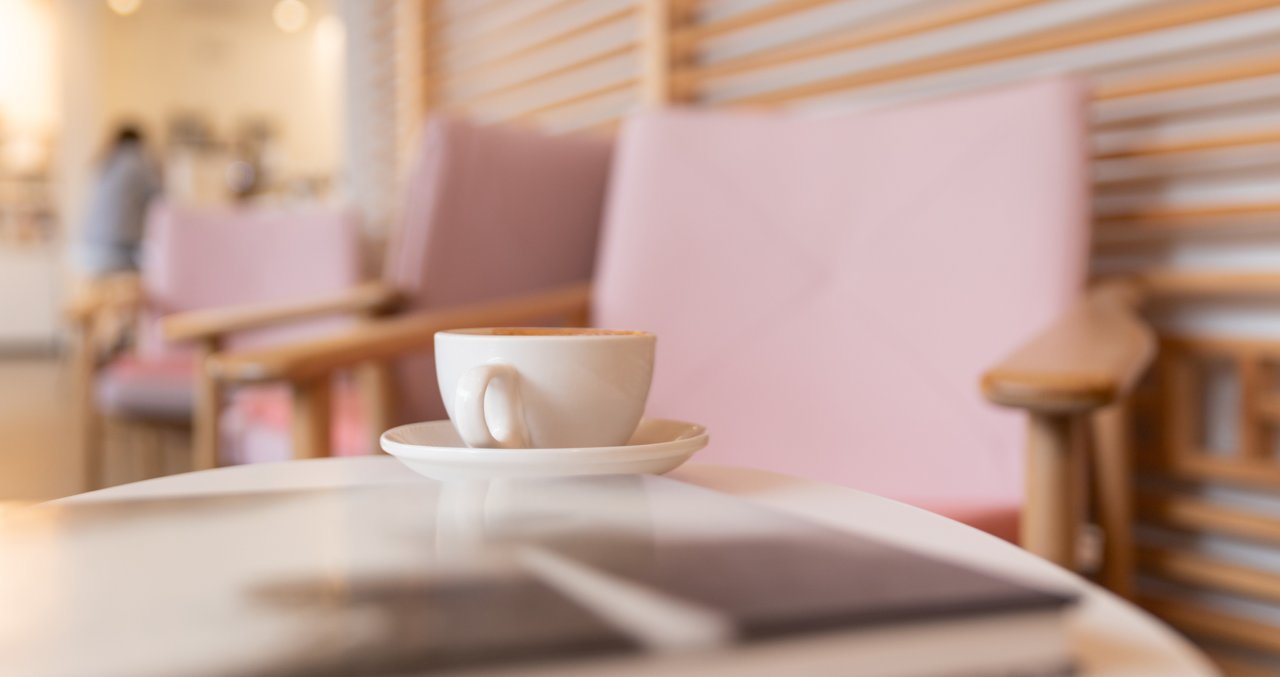The image is a color photograph of a cozy cafe, taken with a fisheye lens which adds a unique distortion to the scene. At the center of the image, a round, short coffee table is prominently featured. Atop the table, a white porcelain saucer holds a bowl-shaped white teacup with a single round handle. The inside of the teacup is brown, possibly containing tea or coffee. Next to the cup, there is a hardcover book that is out of focus, with a black and white photograph on its cover.

Behind the coffee table is a wood-framed chair with a tall back, upholstered in pink fabric and fitted with an orange cushion. Two additional similar chairs are visible towards the left of the image. Beyond these chairs and towards the top left corner, a counter is visible where drinks can be ordered. A person wearing a gray shirt is seen standing at the counter, adding to the bustling atmosphere of the cafe.

The light source appears to be coming from the left, casting a soft glow across the scene. The background features wooden posts running horizontally across the wall, contributing to the cafe's warm and inviting ambiance. The overall style of the photograph is representational realism, capturing a serene and detailed moment within the cafe.